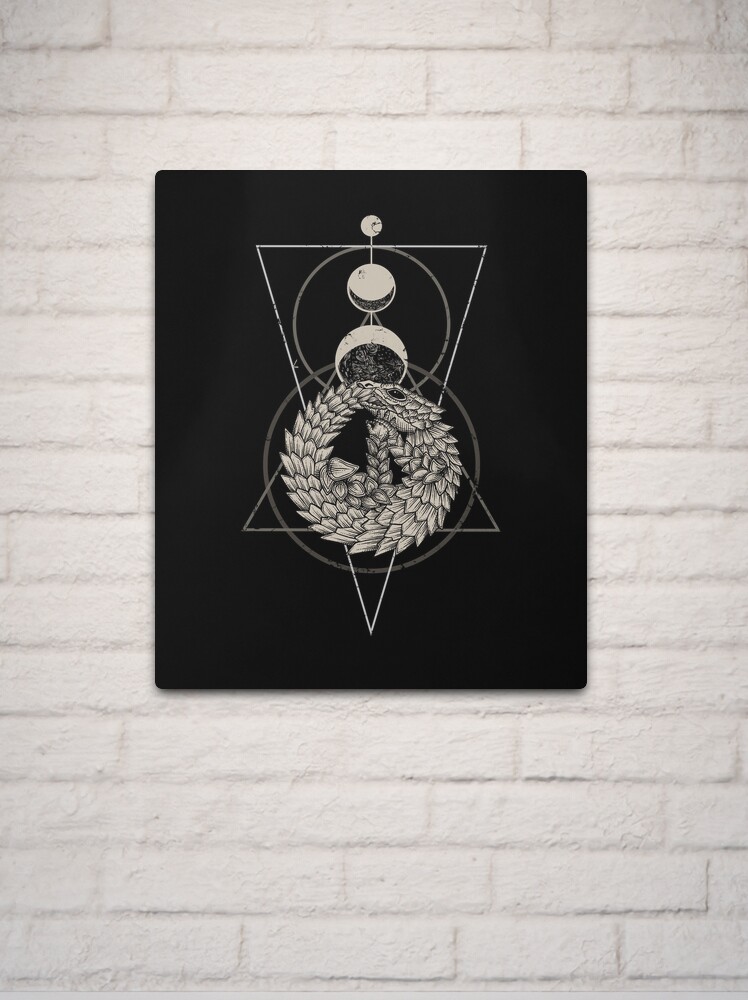This is a detailed photograph of an abstract artwork hanging on a white painted brick wall. The artwork is displayed in portrait orientation and features a solid black canvas. The design on the canvas is predominantly white with some brownish hues, crafted in a geometric and somewhat organic style. At the top of the artwork is a small, shiny, metallic-looking circle casting a shadow. Beneath this is a larger circle, part white and part black, resembling a crescent moon with the black portion at the bottom. Below this is an even larger circle with the crescent moon shape inverted, facing downwards. 

Central to the composition are two overlapping triangles: an isosceles triangle with its base at the top, pointing downwards, and an equilateral triangle below it, pointing upwards. Where these triangles intersect, there is a brownish circle encircling the area. Within the larger triangle is a grayish circle. At the very center of the artwork is a detailed depiction of a snake or dragon curled around itself, its scales ornate and almost leaf-like, creating a sense of movement and texture. The head of this creature is positioned at the top and oriented towards the right, contributing to the mystical and intricate nature of the piece.